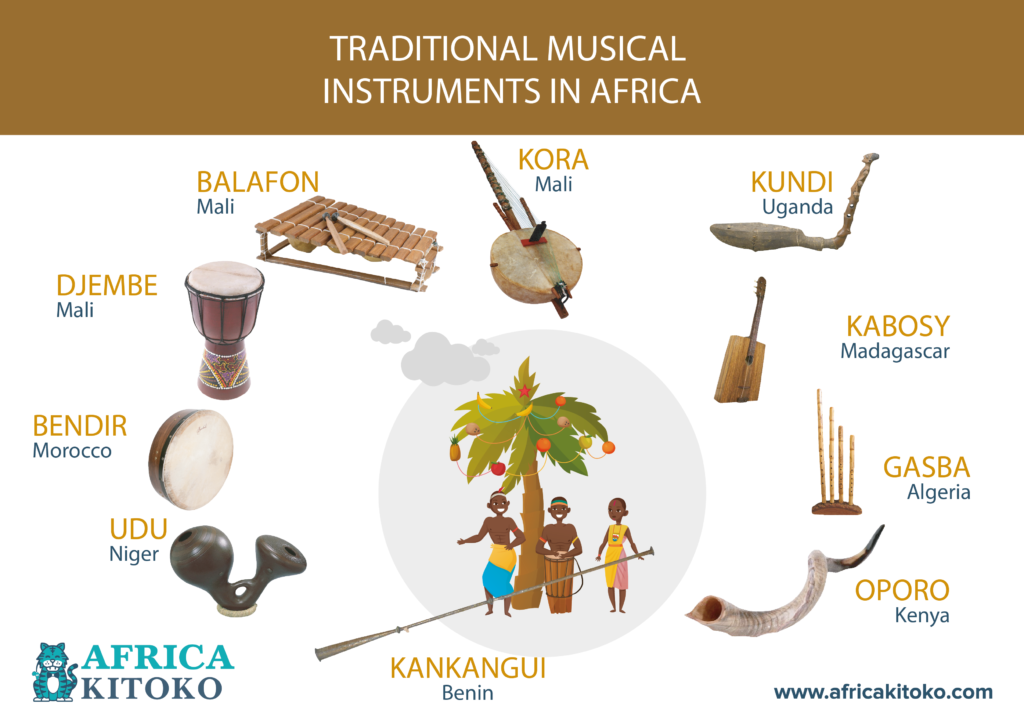This detailed image titled "Traditional Musical Instruments in Africa" features a central scene of three individuals engaging with traditional African culture underneath a whimsical palm tree adorned with pineapples and various other fruits. One person is playing a drum, another is dancing, and the third is holding an elongated instrument, which might be a wind instrument although it is not held to her lips. The image is branded with the "Africa Kitoko" logo in the bottom left, accompanied by a distinctive blue tiger.

Encircling this central vignette are photographs of nine distinct traditional African instruments, each labeled with its name and country of origin. Starting from the lower left and moving clockwise:
1. **Udu from Niger**: Appears to be an instrument fashioned from a gourd, recognized often for its clay pot-like structure.
2. **Bandir from Morocco**: A larger frame drum resembling a tambourine without the jingles.
3. **Djembe from Mali**: A well-known goblet-shaped wooden drum, played with bare hands.
4. **Balafon from Mali**: A wooden xylophone characterized by resonating gourds beneath its slats.
5. **Kora from Mali**: A stringed instrument akin to a harp-lute, notable for its large calabash base.
6. **Kundi from Uganda**: A stringed instrument with a distinctly bent neck.
7. **Kabozi from Madagascar**: A boxy, guitar-like string instrument, often made from wood.
8. **Gasba from Algeria**: Likely a wind instrument with an uncertain structure involving bass sticks.
9. **Oporo from Kenya**: An instrument resembling an ibex horn, used as a wind instrument. 

Each element combines to deliver a comprehensive visual representation of African musical heritage and the rich diversity of its traditional instruments.